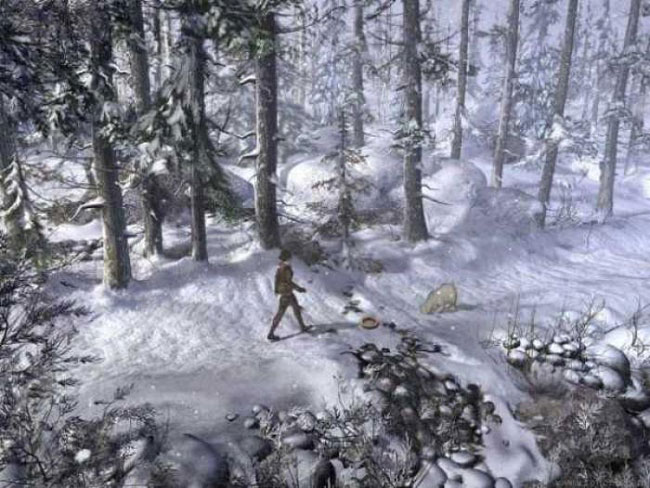The image appears to be a screen capture from a video game, likely a point-and-click adventure possibly set in Siberia. The scene is set within a snowy woodland, characterized by tall trees with a mix of snow-covered pine needles and bare branches. Thick snow blankets the ground, forming larger and smaller piles, while round, small pebbles, rocks, and twigs are scattered across the forest floor. In the center of this image, a person—the main character—is depicted wearing brown pants, a brown jacket, and a hat, stepping forward through the snow. Beside them on the ground, there appears to be an object resembling a bowl. To the right of this figure is a mysterious creature, possibly a polar bear cub or a dog, with its head sticking partly into the snow. The atmospheric details, such as the lack of visible footprints and the snow-laden trees, contribute to the immersive, wintry setting.